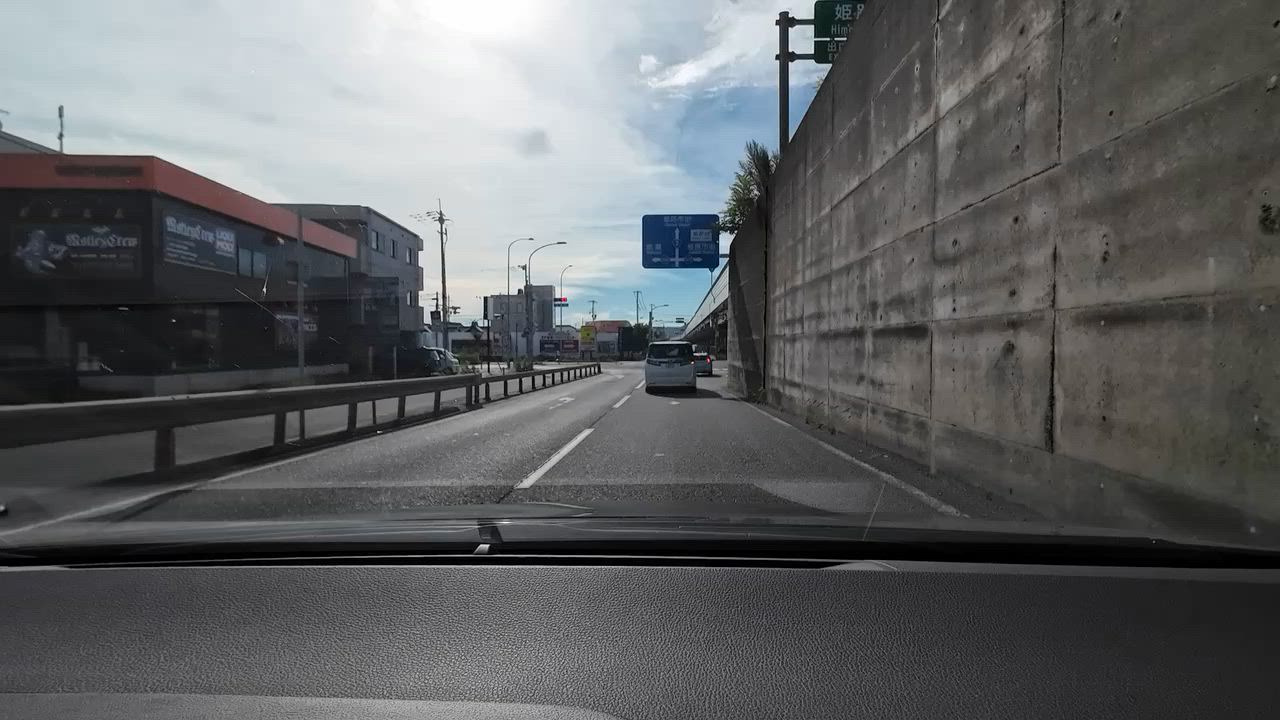This outdoor photograph captures a detailed street view from the perspective of a car's dashboard, visible at the bottom. The image showcases a divided urban highway with four lanes; two lanes in each direction separated by a metal median barrier. To the right, there is a grayish concrete sound barrier wall, with a blurred green road sign above it indicating the route, although the text on the sign isn’t readable. Moving further into the image, the lanes on the right curve slightly to the left. Directly ahead, another vehicle, likely a white minivan, travels in the same direction. On the left side of the roadway sits a low metal fence and a series of urban structures, including a large two-story black building with a distinctive red band at its top and several tan and brown buildings further back. The horizon reveals more commercial and industrial buildings along with streetlights. The sky above is a mix of blue with clouds predominantly occupying the left portion, giving the scene an overcast appearance.